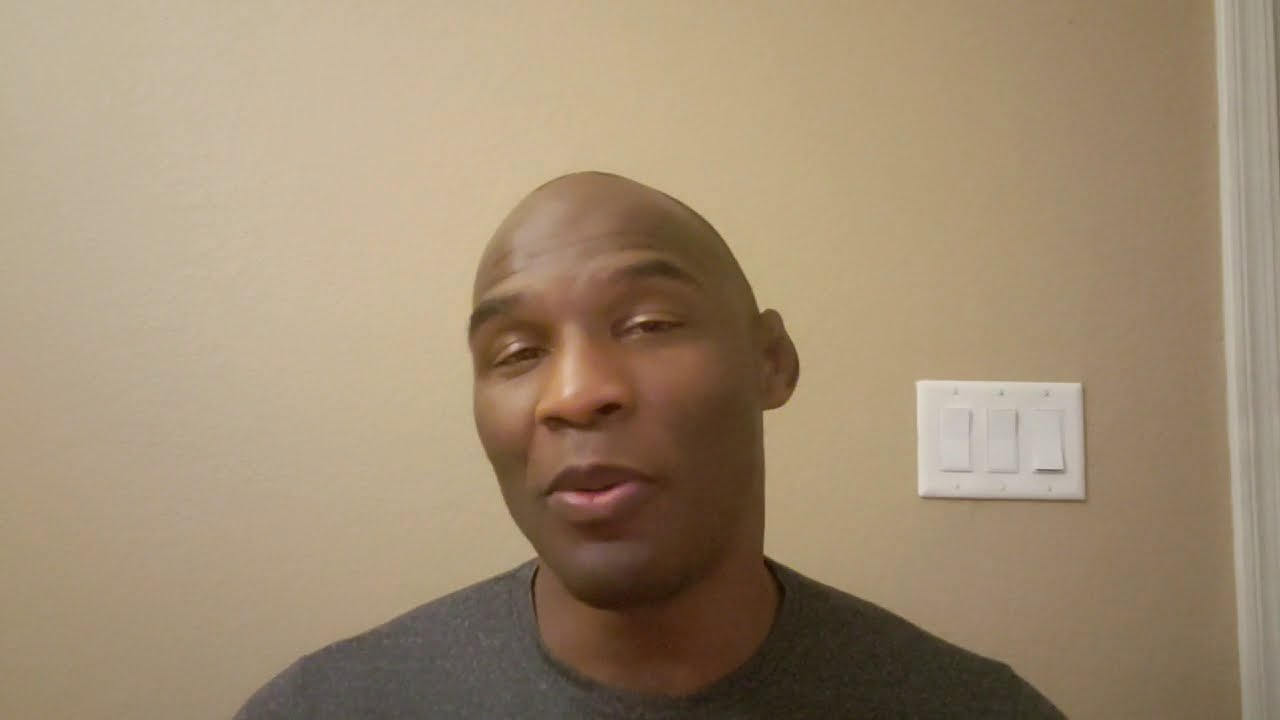The image captures a young, bald, black man, who is centered in the photograph, gazing directly at the camera with a faint smirk. His dark eyebrows contrast with his partially closed eyes, which reveal just a sliver of his pupils, giving him a slightly tired or relaxed appearance. His lips are closed but you can notice a subtle hint of pink on his bottom lip. One of his ears, slightly resembling a cauliflower ear, is visible on the viewer's right side. He's dressed in a simple gray t-shirt, and the background is a cream-colored wall that transitions from lighter on the left to slightly darker on the right. Prominently featured behind him is a rectangular white switch plate with three button-style light switches. Additionally, the trim of a doorway can be seen on the far right side of the image, subtly slanted inward towards the left. This photo, possibly a selfie, captures the man alone against this plain backdrop.